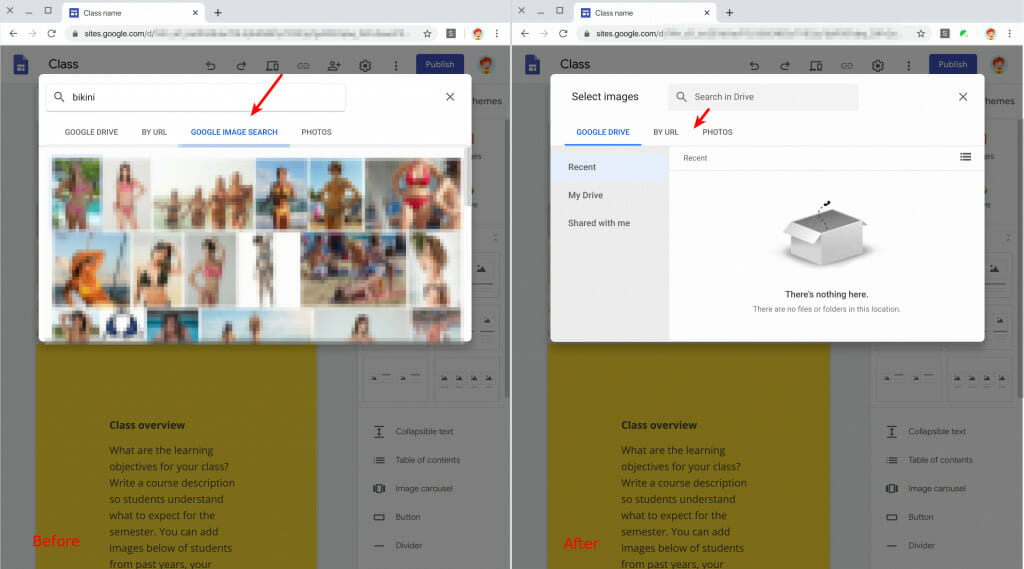The image consists of two screenshots of a web page open in a browser tab with the URL "site.google.com." The first screenshot showcases a search field with several options listed: "Beginning," "Categories," "Google Drive," "By URL," and "Google Image Search." A red arrow is prominently pointing towards "Google Image Search," indicating the element of interest. 

The second screenshot features another section of the webpage where a red arrow points towards the "By URL" option. Additional text present in this screenshot reads: "Recent," "My Drive," "Shared with Me," and a message that says, "There are no files or folders in this location."

Below this, an instructional section titled "Class Overview" asks, "What are the learning objectives for your class?" It advises writing a course description to help students understand what to expect for the semester. It also suggests adding images of students from previous years.